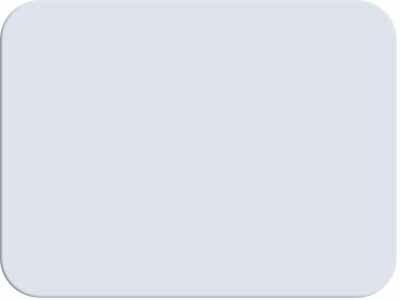A close-up image showcases a button element on a web browser, meticulously cropped and zoomed in to reveal its intricate details. The button is a light gray rectangle with rounded edges, slightly wider than it is tall, giving it a balanced yet functional appearance. The surface of the button is uniformly light gray, contributing to its minimalist design. On the left side, a subtle shadow effect introduces a sense of depth and dimension, suggesting that the button can be pressed. This shadow effect is more pronounced on the left, creating the illusion of an off-angled light source or camera. The right side lacks this shadow, appearing marginally lighter, which enhances the perception of depth and the button's three-dimensional form. The image is somewhat pixelated, reinforcing the impression that it has been significantly zoomed in, adding a touch of digital texture to the otherwise simple interface component.